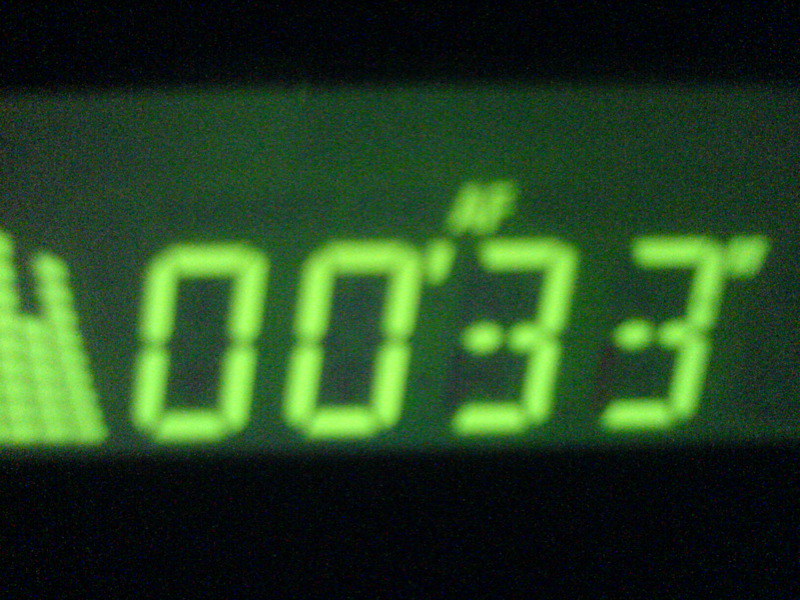The image is a blurry photograph of a digital interface or LED screen with a dark green background and some splotchy lighter green areas. The screen features old-fashioned LED-style numbers in neon lime green that read "0033," with an "AF" above the second three, positioned at the top right of the comma. On the left side, there is a symbol resembling sound waves or a crown made of small green dots, slanting towards the left. The rectangular-shaped interface has a dark, nearly black border that blends into the green screen, especially at the top, due to the blurriness of the picture. Black lines are present at the top and bottom of the screen, with the bottom one being thicker and wider.